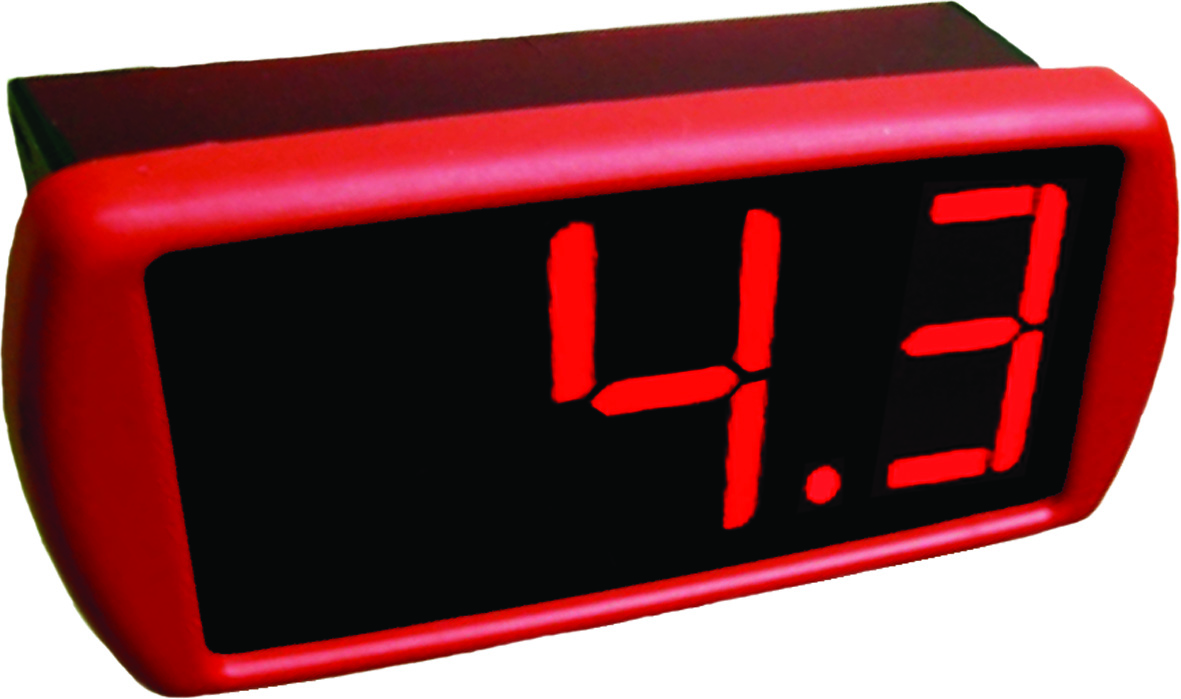The image features a digital clock with a red outline surrounding a black rectangular display. The time shown is '4.3,' with the number '4' constructed from four distinct, linear segments and '3' made up of five separate linear segments, giving them a geometric appearance rather than a curved one. Above the digital display, there's a brown wooden element that extends across the top of the clock, adding a rustic touch to the otherwise modern device.